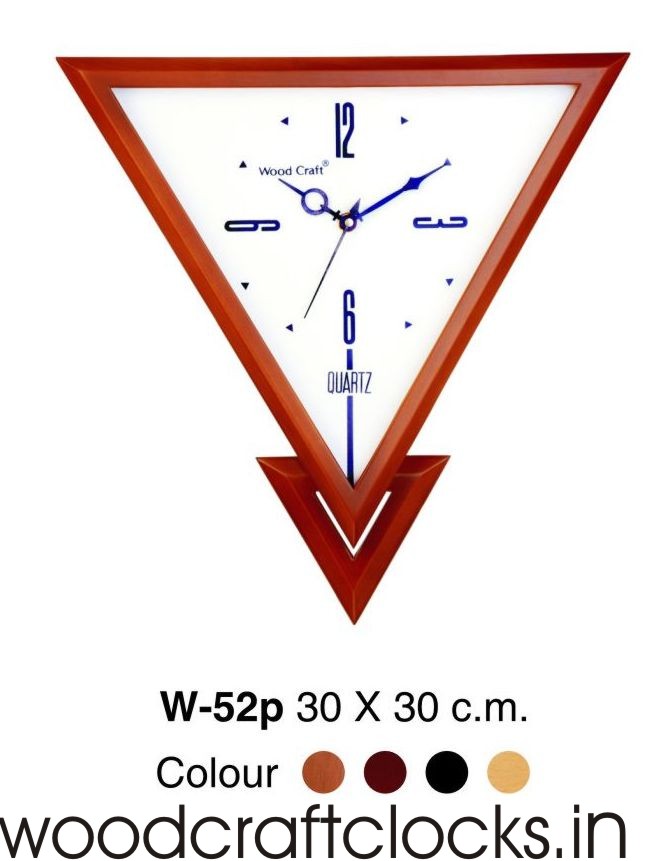This advertisement showcases a unique wall clock designed in the shape of an upside-down triangle with a smaller triangle at its tip, both made of wood in varied shades of brown. The larger triangle forms the main body of the clock with a white face, while the smaller triangle, fittingly darker, resides at the bottom point. The clock face features narrow, vertically aligned numbers at 12 and 6, and horizontally aligned 3 and 9, all in blue. The remaining hours are marked by small triangles. An elegant blue hour hand resembling a key, a blue minute hand with a diamond-like center, and a blue second hand pointing near the 7 o'clock mark, indicate the time set to 10:10 and approximately 35 seconds. Prominent blue inscriptions include "woodcraft" to the right and "quartz" beneath the 6. Below the main clock, in large black print, are specifications: "W-52P, 30 by 30 cm, color" accompanied by color dots denoting light brown, dark brown, black, and tan. The advertisement concludes with "woodcraftclocks.in" indicating the product's craftsmanship and origin. The background of the image is stark white, accentuating the design and colors of the clock.